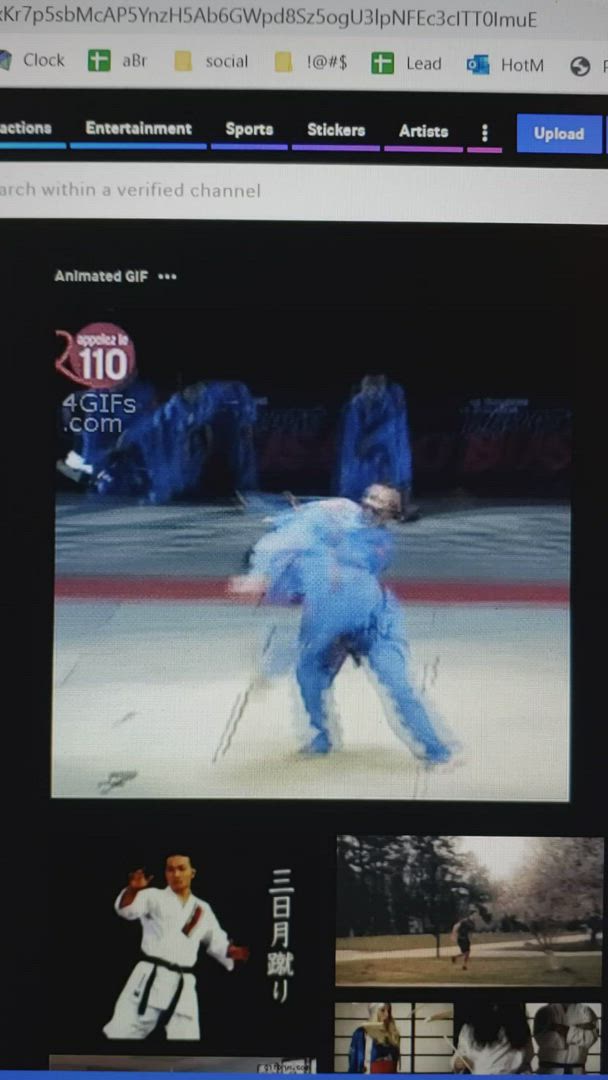The image consists of a collage with multiple photographs presented in a vertical arrangement. The topmost image, sourced from GIFs.com, is notably blurry, making it difficult to discern specific details. From what can be observed, a man, appearing to wear denim overalls, stands on a white tiled floor. The peculiar aspect of this image is that his body seems to lean as if he's on the verge of falling, and rather unusually, his head is attached to his upper arm instead of his shoulders.

The midsection of the collage contains two side-by-side images against a black background. On the left, a martial artist is depicted, seemingly of Asian descent. He is dressed in a traditional white robe with a black belt, poised with his arms and body in a stance that suggests he is about to perform a martial arts move.

On the right side of this midsection and directly beneath the top image, there's a separate photo showing a person walking across a grassy area in what appears to be a park. Behind this individual, there is a walkway followed by more grass and some trees, suggesting a serene, natural environment.

The bottommost part of the collage features another photograph that is dimly visible due to its small size, making it hard to discern any specific details.